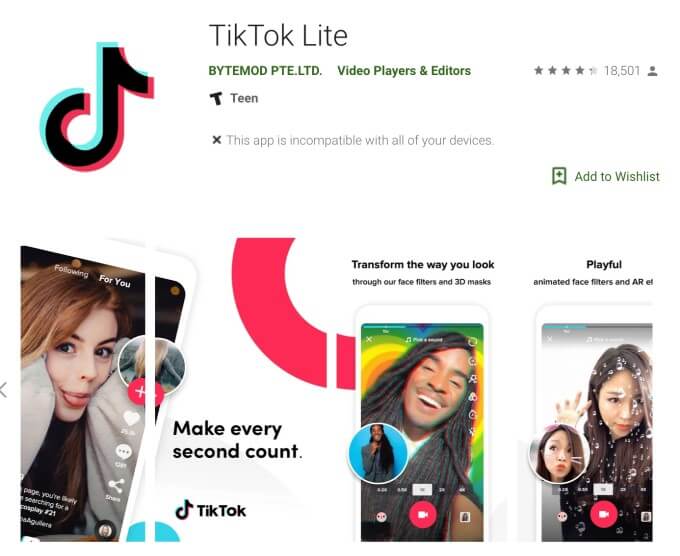Under the category of webpages, featuring a clean white background, the image showcases the app "TikTok Lite" prominently at the top. The app is developed by ByteMod PTE and falls under the category of video players and editors. It has received a solid four-star rating from 18,501 reviewers and is rated T for Teen. A note indicates that the app is incompatible with all of your devices. A recognizable TikTok logo is displayed as well. 

At the bottom of the image, three phone screenshots are displayed:

- The rightmost screenshot features an Asian woman surrounded by whimsical bubbles, set against a gray background.
- The central screenshot captures an African American man with long dreads and a mustache, laughing joyfully. His background is a vibrant, psychedelic swirl of oranges, greens, yellows, and blues.
- The leftmost screenshot depicts a young woman wearing a white jacket over a black shirt. She has striking red hair with blonde streaks.

Each image vividly showcases diverse content and the lively community within the TikTok Lite app.